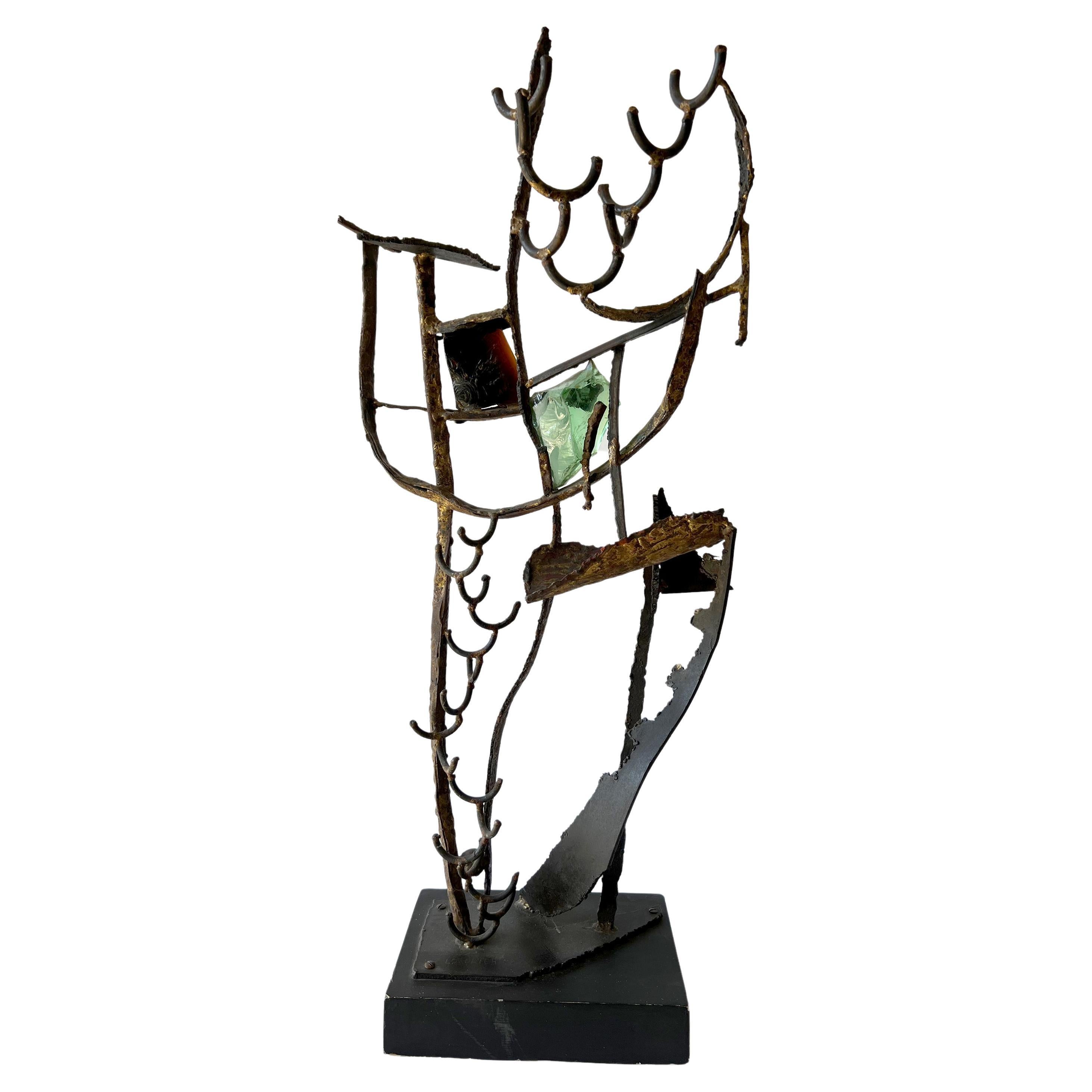The image features a tall, intricate sculpture set against a white background, displayed on a black square stand. The sculpture is constructed primarily of metal with elements of glass and wood interspersed throughout. It consists of several thin, branch-like protrusions with U-shaped curves, some of which are reminiscent of antlers or organic forms. These protrusions rise up in a somewhat circular, twisting pattern. Near the center of the artwork, there is a piece of green glass or a transparent rock, as well as a darker, reddish-black rock. The combination of these mixed media elements—including metal, glass, and wood—creates a complex, abstract form that is visually striking. Overall, the piece is a dark-colored assemblage, devoid of any writing or figures, emphasizing its abstract and artistic nature.